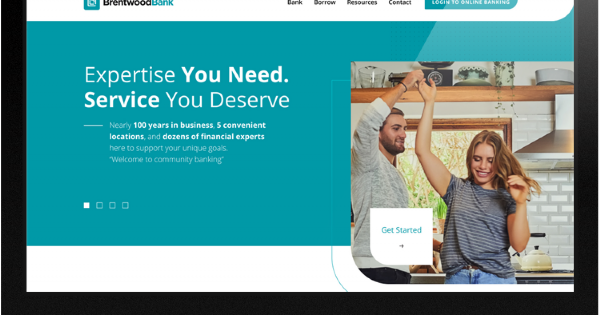Brentwood Bank’s website features an elegant and modern design with a color scheme of black, white, and turquoise. The homepage prominently displays the tagline, "Experience you need, service you deserve." To the right of this text, there is an image of a joyful couple dancing. Beneath the tagline, an additional line reads, "100 years in business, five convenient locations, dozens of financial experts." Positioned above the image is a turquoise "Get Started" button inviting user engagement.

The top of the webpage includes navigation options labeled "Bank," "Borrow," "Resources," and "Contact," alongside a login area for customers. The banner also features the bank's name, Brentwood Bank, accompanied by a turquoise and white logo, which is somewhat abstract and subtle.

Notably, the homepage contains a dynamic slideshow feature, allowing visitors to view various slides by clicking navigation buttons at the bottom of the screen.